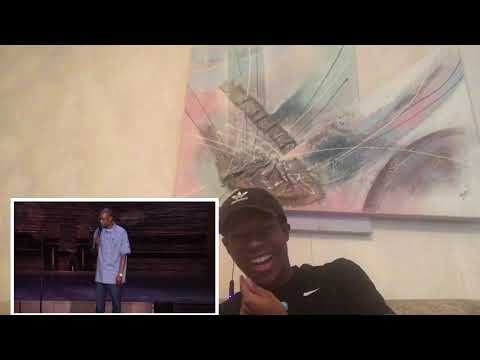The image features a black man sitting on a couch against a white or beige wall, reacting to a stand-up comedy video. He is wearing a black long-sleeved Nike shirt and an Adidas hat, laughing hysterically. Behind him hangs a watercolor painting in pastel hues of teal and pink. The video he is recording himself watching is displayed in the bottom left corner of the image. It shows another black man on stage, dressed in a blue short-sleeved button-down shirt and jeans, holding a microphone and wearing a watch on his left wrist. The scene captures the essence of a humorous moment as conveyed by the man’s joyful reaction.